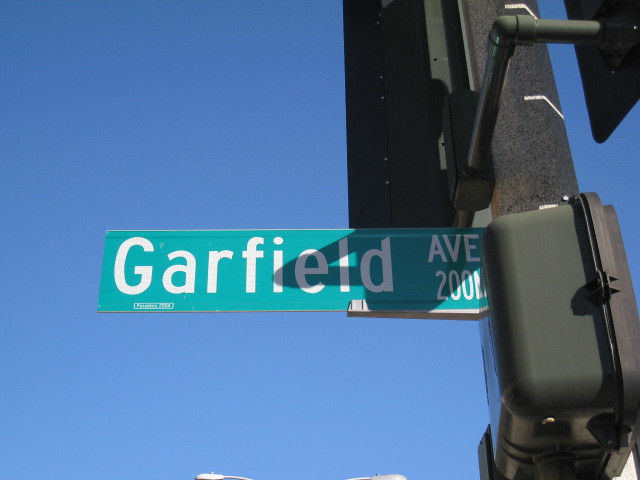The photograph captures a sunny outdoor scene against a clear, bright blue sky devoid of clouds. Dominating the image is a solid black traffic light pole with various black attachments protruding from it, though their specific functions are unclear. Mounted on this pole is a green street sign displaying "GARFIELD AVE" in white capital letters, indicating Garfield Avenue. Adjacent to this is the street number, "200," though part of it is obscured. Below the street sign, there is a small dark gray box with a black front, possibly a pedestrian signal box for crosswalk instructions, though the details are not fully visible. The setting appears to be the 200 block of Garfield Avenue.